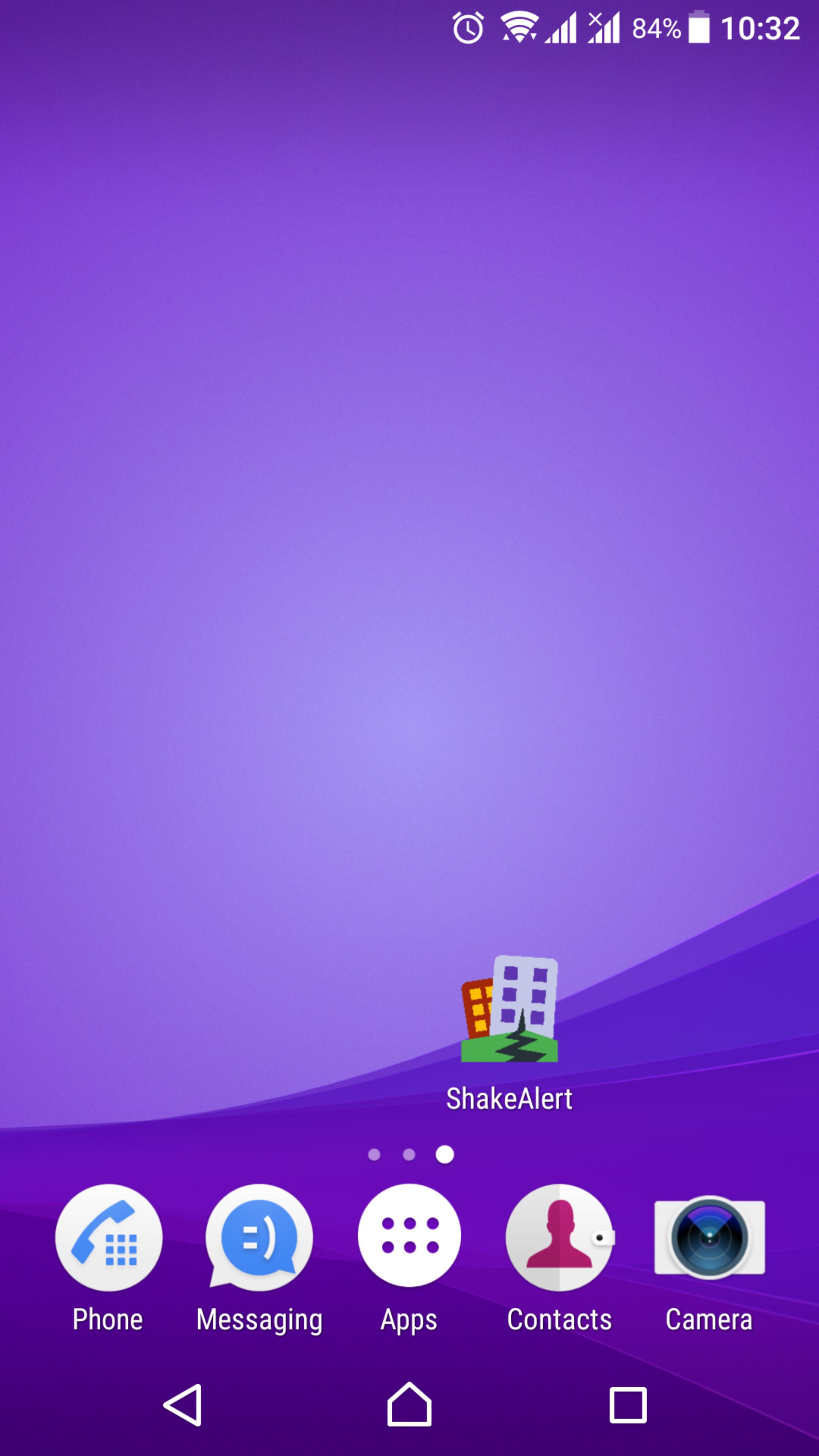The image features a gradient background transitioning smoothly from a rich purple at the top to a lighter purple, followed by dark purple, and gradually blending into a bluish hue. The bottom left corner of the background is particularly dark purple. This image, a snapshot from a smartphone, showcases various details and elements.

In the bottom-right section of the screen, there is an app icon for ShakeAlert. The text "ShakeAlert" is prominently written in white. The icon itself depicts two buildings: a gray building with purple windows in the foreground and a red building with yellow windows in the background. The foreground building and the ground below it are shown with visible cracks, symbolizing the app’s function of alerting users to earthquakes or ground shaking events.

Additionally, there are several app icons displayed in a row at the bottom of the screen:

1. A Phone app icon featuring a white and blue glyph.
2. A Messaging app icon also with a white and blue glyph.
3. In the center, there is an App Drawer icon, a white circle dotted with six purple dots arranged in a grid pattern.
4. The Contacts app icon, predominantly white with a pink accent.
5. The Camera app icon, which is white, showcasing a camera lens graphic that combines purple and blue hues.

The composition of the image blends vibrant colors with practical icons, creating a visually appealing and informative smartphone interface.